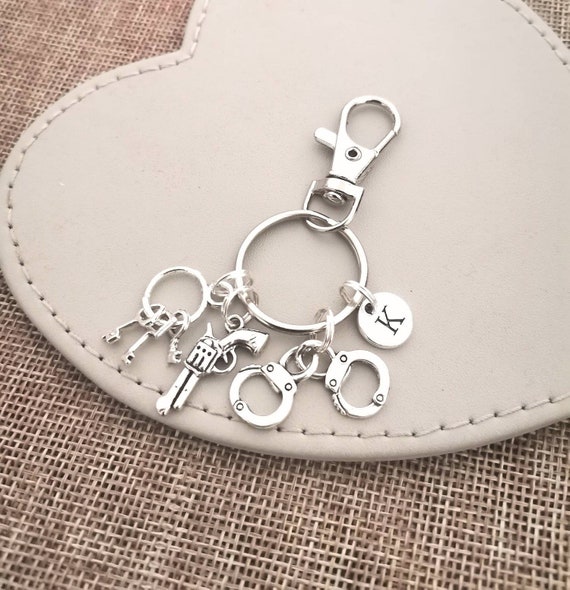The image showcases a close-up of a keychain adorned with several small, silver-metal charms including a set of prison keys, a handgun, handcuffs, and a circular tag with the letter 'K'. These charms are intricately attached to a silver key ring. The keychain is artfully laid on top of a light pink leather heart, which is positioned diagonally from the top right corner and threaded with fabric. This fabric appears to be a rough, light-brown crosswork, almost straw-like in texture. The background consists of neutral, washed-out colors, contributing to a soft and balanced aesthetic. The overall setting is bright with natural lighting, highlighting the shine of the silver charms against the muted tones of the heart and fabric. The presentation suggests a product photograph aimed at showcasing the keychain's detailed design.